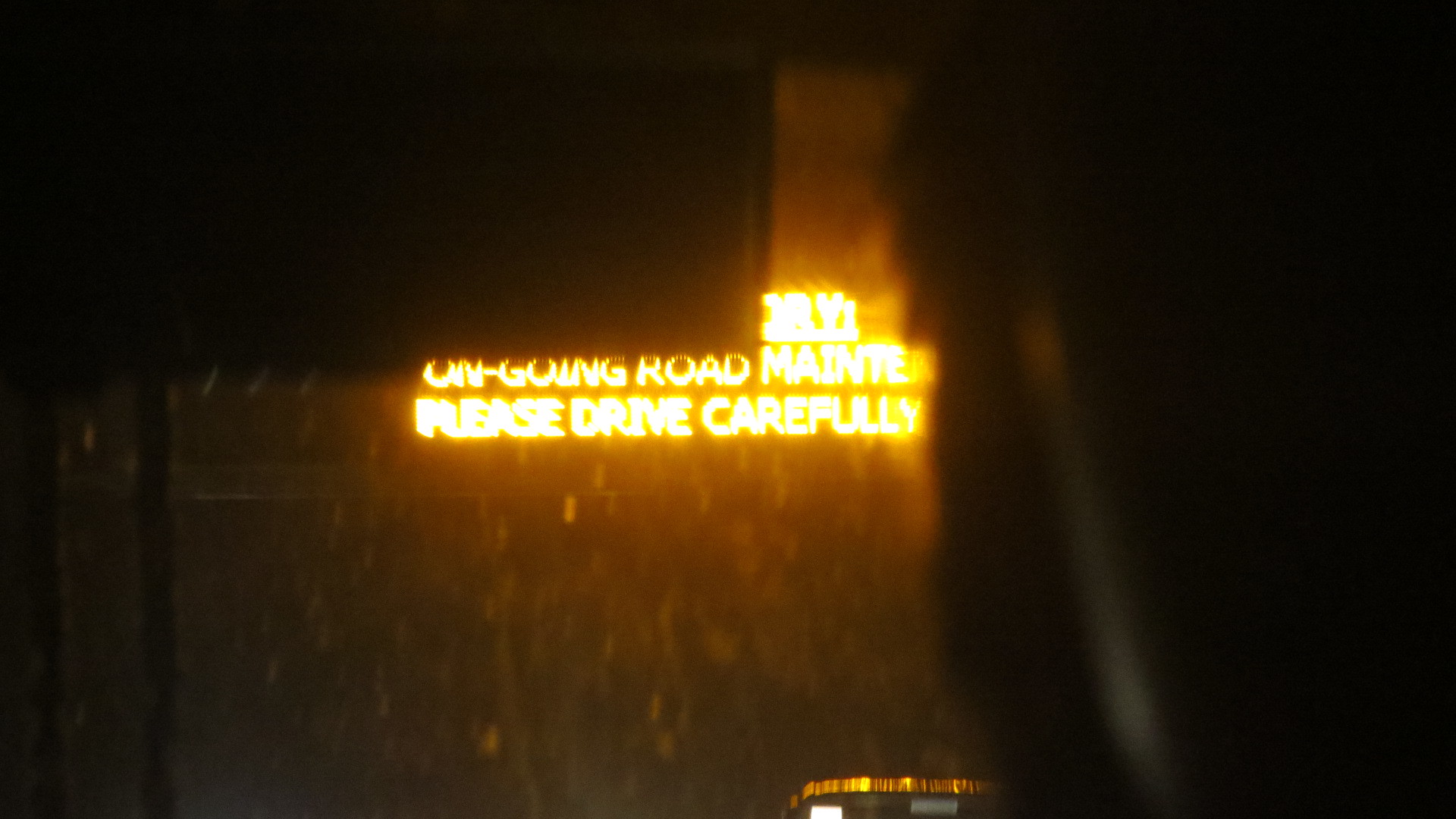This color photograph exhibits a slightly blurred aesthetic, contributing to an enigmatic atmosphere. In the top left corner, an indistinguishable object, possibly a seat, can be seen. Dominating the lower section is a dark wooden floor, juxtaposed against a black leather bench situated on the right. The floor is intriguingly lit, creating an illusion of imposed writing that reads: "Ongoing road, main, please drive carefully." This adds to the photograph's surreal quality, making it unclear whether the scene is set indoors or outdoors. A highlighted gold band accentuates the bottom of the image, enhancing its overall mystical and reflective ambiance.